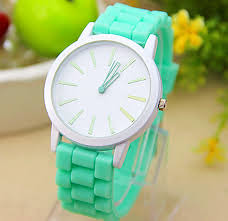The image depicts a lady's wristwatch prominently displayed on a clear perspex holder, positioned on a beige table. The watch features a silver-toned bezel and a white face with green and yellow hour indicators, devoid of any numerals. The mint green hands match the linked band, which appears to be made of silicone. The band mimics the style of traditional metal links but in a rubber-like material. Observably, the watch is clasped at the back, and the face slightly tilted to the left. In the blurred background, a bowl containing a green apple is visible, along with a yellow flower to the right, adding a touch of color and context to the setting.